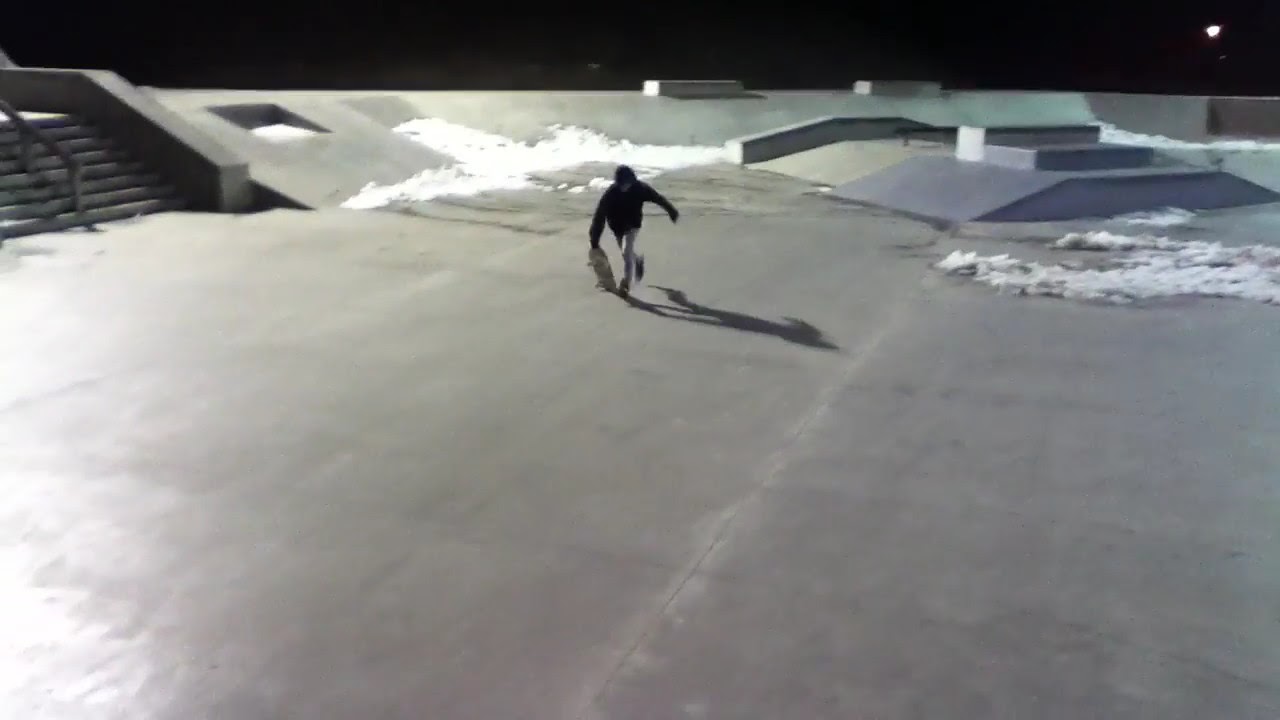In this detailed nighttime scene at an outdoor skate park, illuminated by streetlights, a lone individual is captured in motion, clutching a skateboard in their right hand. The figure is dressed in a black hoodie with the hood up and white pants, and their shadow is cast to their right on the concrete surface that spans most of the park. Snow is scattered across the ground, indicating a winter setting. The skate park features various structures, including ramps, an elevated platform, medians with metal and concrete railings perfect for grinding, and an eight-step staircase with a central railing. The backdrop is a dark, night sky, adding a dramatic contrast to the gray and white tones prevalent in the skate park.